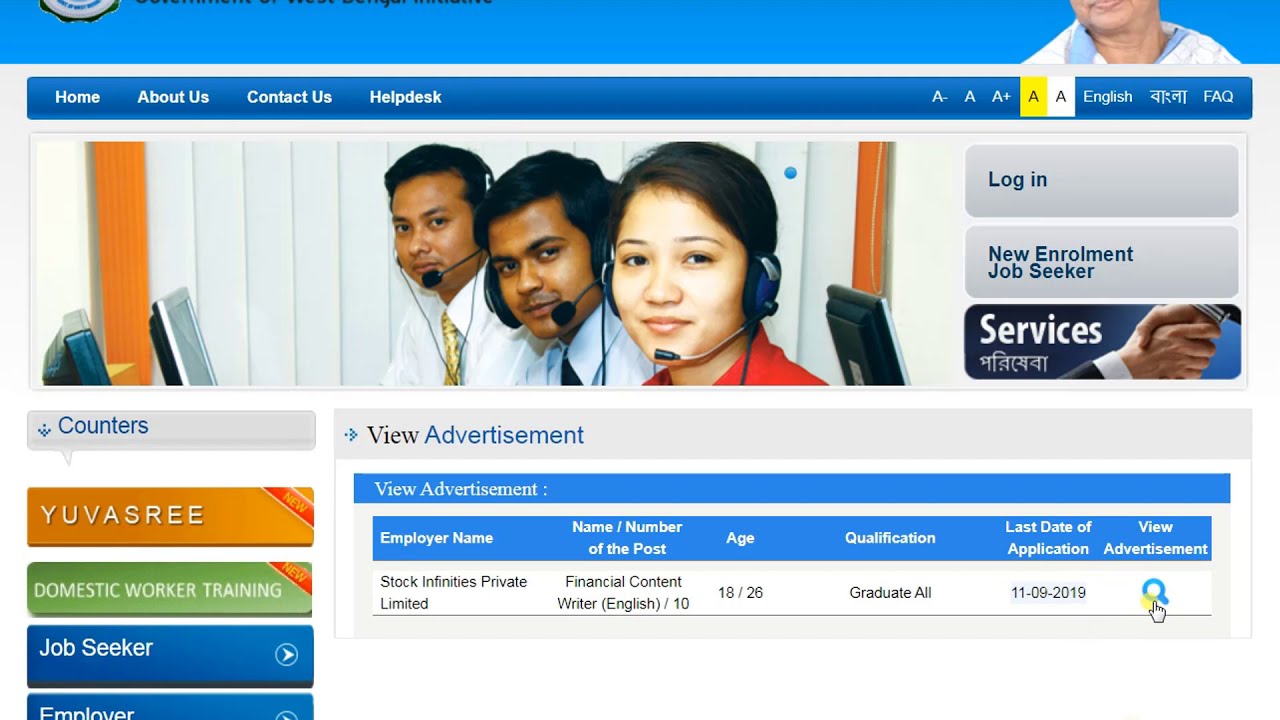The screenshot captures a website interface featuring a prominent blue banner at the top, which includes a navigation tab bar with options: Home, About Us, Contact Us, and Help Desk in white text. Below this banner is an image of three customer service representatives: a woman with brown hair and a red shirt, a man with short black hair in a blue collared shirt and tie, and another man in a white collared shirt with a gold tie. They are wearing headsets with mouthpieces and posing with vertical blinds and computer screens visible behind them. The right side of the interface includes various clickable links such as Login, New Enrollment, Job Seeker, Services, alongside labeled sections like Counters, U of S, Domestic Worker Training, Job Seeker, Employer, and detailed advertisement links mentioning Employer Name, Number of the Post, Age, Qualification, and Last Date of Application. There is also a language selection option and a list of services tabs available for interaction. This detailed and vibrant website layout is filled with various interactive elements designed to engage users immediately upon visiting the page.